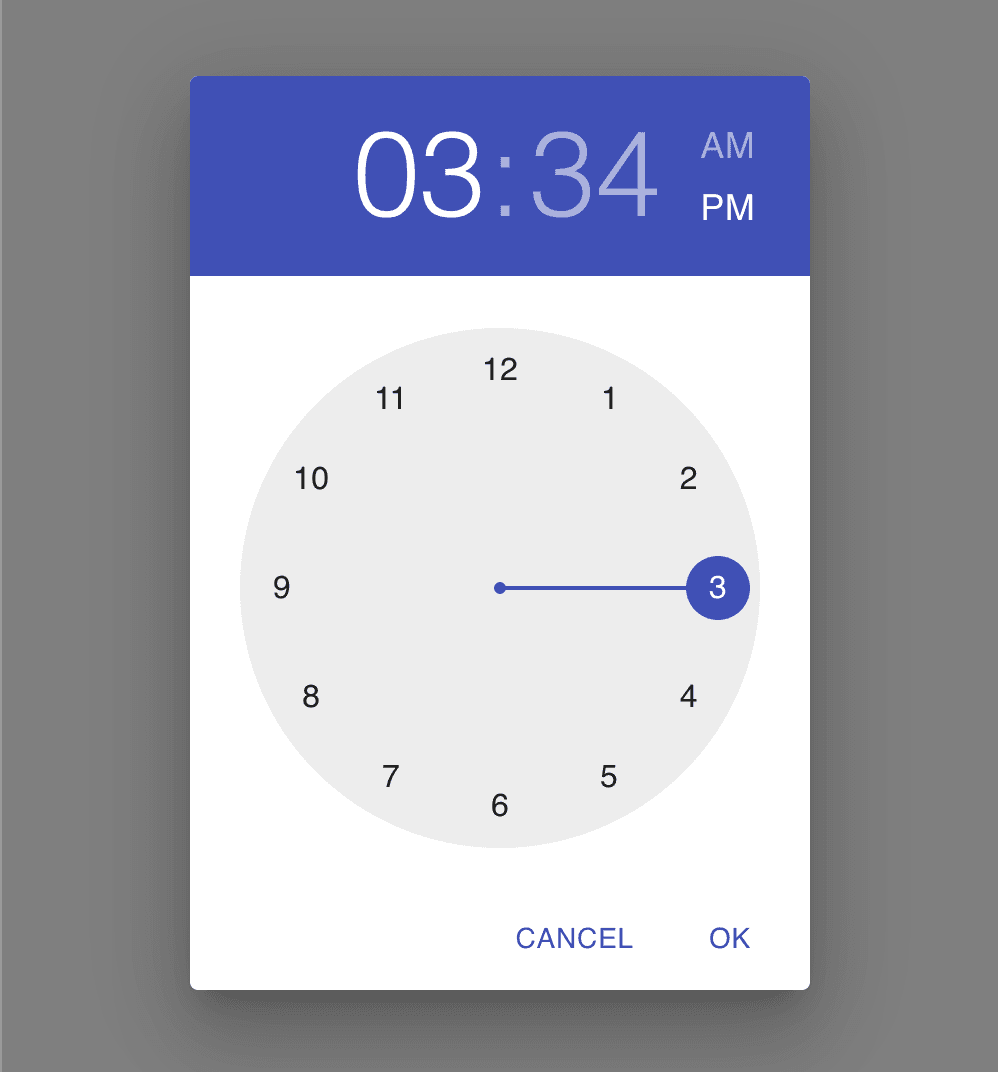The image features a digital clock display set against a gray rectangular background. Superimposed on this background is a white rectangle, with its top portion shaded in blue. The digital time "03:34" is prominently displayed within this blue section. The "03" and the colon are in white, while the "34" is in a lighter blue color. Additionally, "AM" is shown in light blue, while "PM" remains in white, suggesting a selectable option between the two.

Beneath the digital display, a prominent gray circle is centered within the white rectangle. Surrounding this circle are the numbers of a traditional clock face, starting with "12" at the top center. Clockwise, the numbers continue with "1" at a slight right angle from the top, followed by "2" and then "3" at the far right. The sequence continues with "4," "5," and "6" at the bottom center, then "7," "8," "9" on the left, and finally "10" and "11," completing the circle back to "12."

At the bottom of the image, there is a blue rectangular box containing two buttons: "Cancel" and "OK," both also in blue, suggesting user interaction options for setting the time.